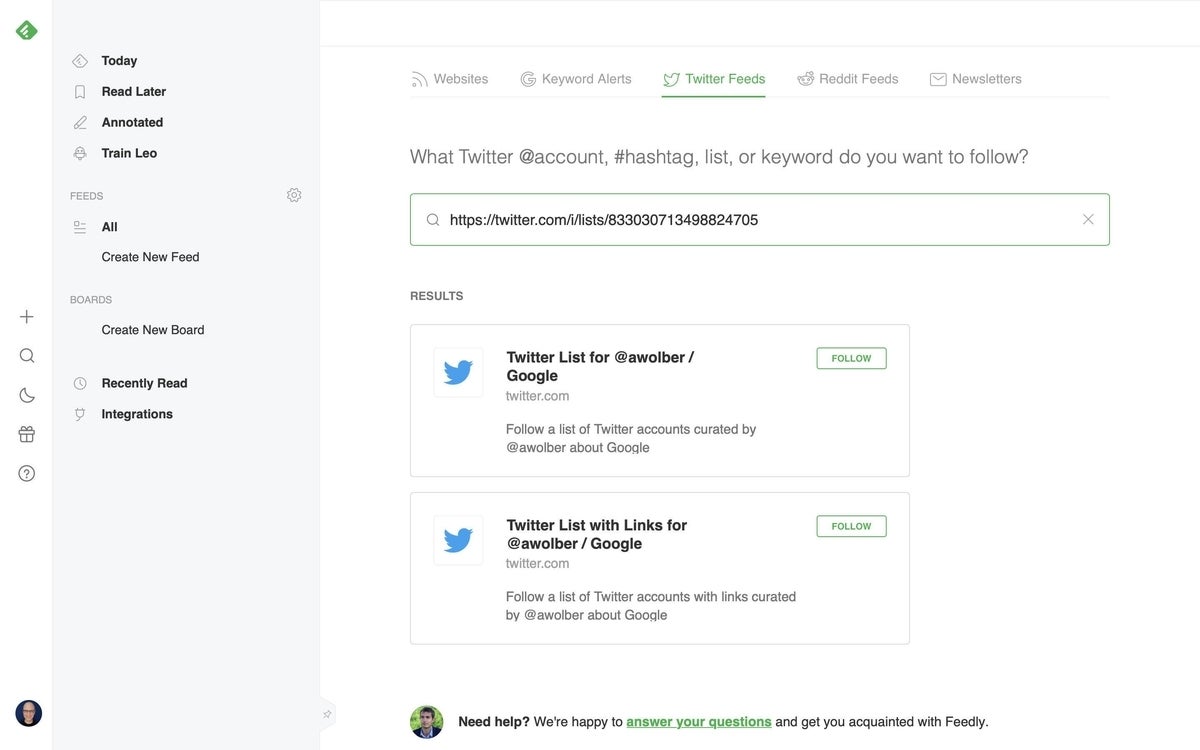The image is a screenshot from an unidentified web page featuring a tool for managing social media, specifically Twitter. The webpage has a white background with a very light gray sidebar on the left side. There is no header at the top, making it impossible to identify the website or the company that owns it.

The main section of the webpage, with its white background, prominently displays a top menu bar with several options labeled "Websites," "Keyword Alerts," "Twitter Feeds," "Reddit Feeds," and "Newsletters," listed from left to right. Beneath this menu bar, a headline written in gray asks, "Which @account, hashtag, list, or keyword do you want to follow?"

Below the headline, there is a rectangular outline containing a web address for a Twitter list: "twitter.com/list/," followed by a long string of numbers. Additionally, two Twitter lists are mentioned. Both are associated with the user "@awobber" and focus on Google-related topics. Each list is accompanied by the classic blue Twitter bird icon, indicative of the time when the platform was still branded as Twitter. The listed items read, "Twitter lists for @awobber/Google" and "A list with links for @awobber/Google."